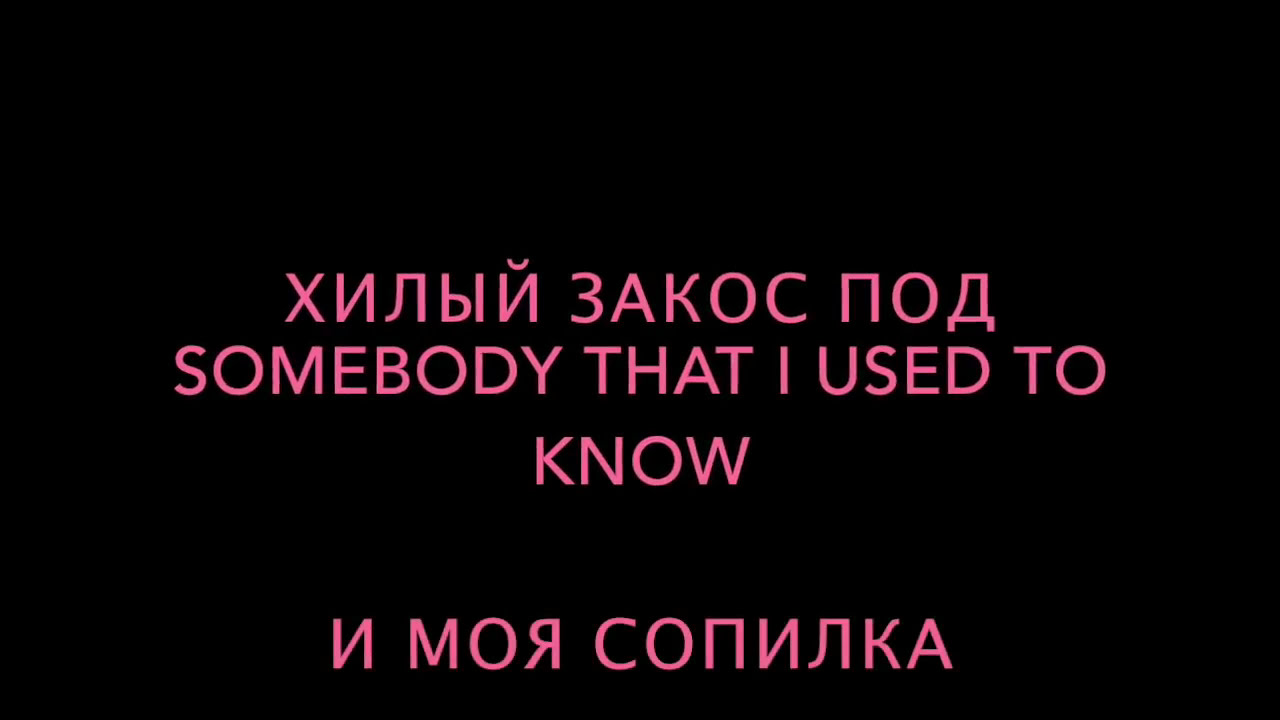The image is a digital screenshot featuring a solid black rectangular background that creates a featureless, empty void effect around the centrally placed text. The rectangle’s top and bottom edges are significantly longer than the left and right edges, effectively doubling their size. In the center of this void, there are four lines of text. The first line is composed of three words in Cyrillic script. The second line, in bubblegum pink text, reads "somebody that I used to." The third line, also in pink text, reads "no," though with a space between "k" and "now," hence it appears as "k no w." The fourth and final line, again in Cyrillic script, contains three more words. The centered alignment of the text emphasizes its presence against the stark black background, making it appear as though it is floating in mid-air.